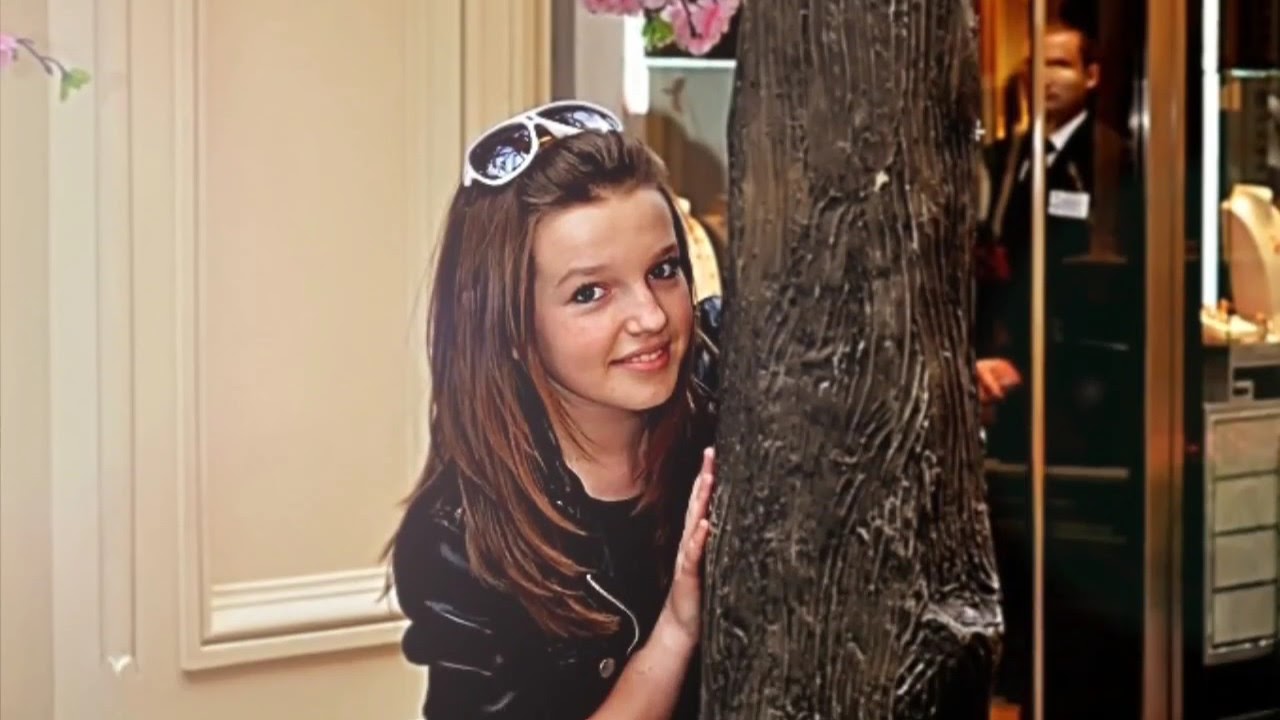In this detailed photograph, a young girl is seen inside a room, standing slightly bent behind a large, vertically standing, brown wooden object that resembles a tree trunk. The girl, with her long, straight, thick brown hair pulled back by a pair of sunglasses resting on her head, joyfully smiles at the viewers. She is dressed in a black jacket with visible zippers and buttons, and she has both hands placed on the trunk. Her face and upper body are clearly visible. 

Behind her, there is a cream or beige-colored door or cabinet. To the right, through a glass door or window, there's a man dressed in a formal black and white suit with a tie, possibly wearing a name tag, standing in a stern posture with his hands folded in front of him. The room also features a tan wall with leaf-like moldings and panel settings. Additionally, subtle details like some pink and green flowers can be seen cascading from the top center and left top of the photograph. On the right side, in the background, a white piece of furniture and possibly a mannequin or model are also visible, adding to the complexity and interest of the scene.